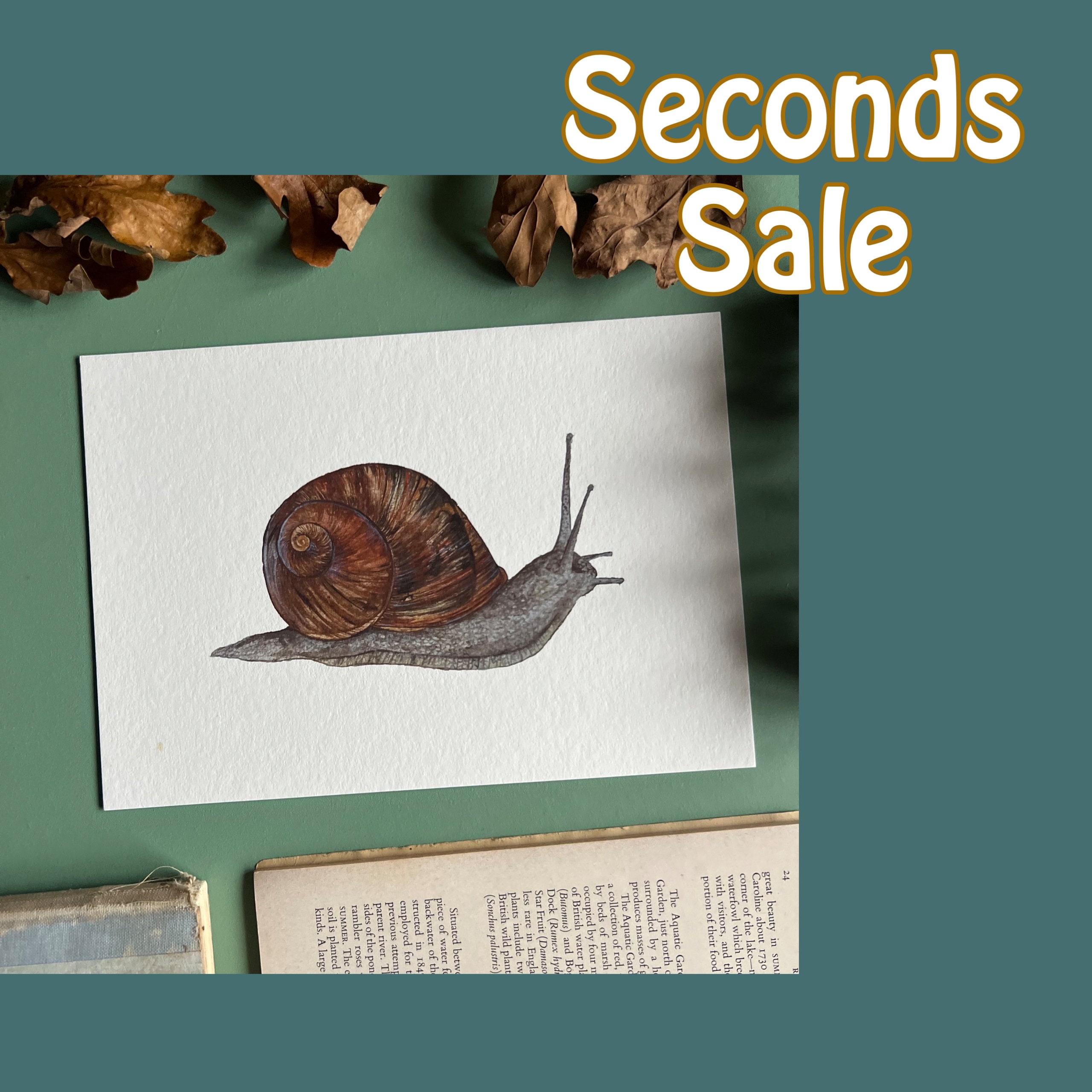The image is a detailed, square poster with a predominantly teal and grayish-aqua background. At the center, there is a white sheet of paper featuring a meticulously drawn snail. The snail's body is gray with large antennae and a small black eye, while its shell is a brown spiral with subtle yellow shading. Above the snail, the background transitions to a greenish hue adorned with old, crunchy leaves. Below the snail, there's an open book, revealing page 24 with visible writing, and another closed book with a worn binding. In the upper right section of the poster, the phrase "SECONDS SALE" is displayed in a whimsical, ruby-colored font. The overall scene is further framed by splashes of dark aqua, tying all elements together in a cohesive, artistic presentation.